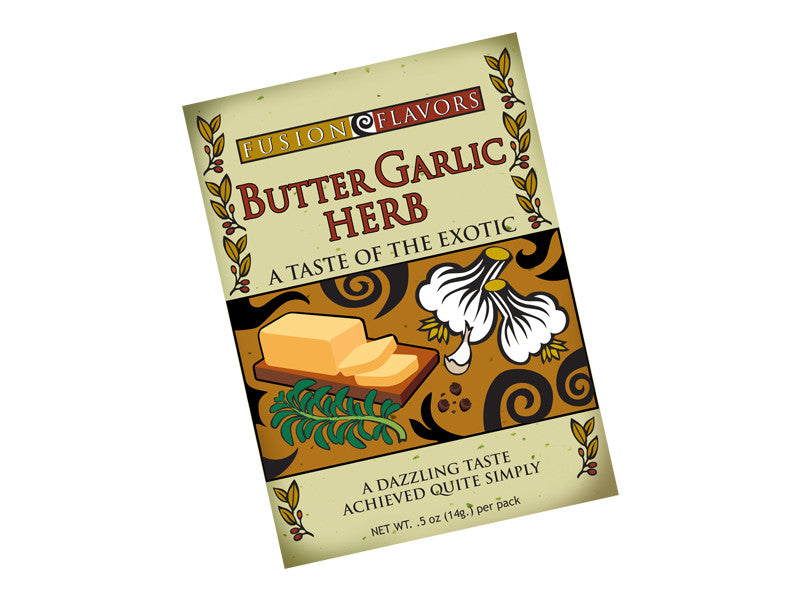The image features a tilted package cover, positioned diagonally towards the center with a slight inclination to the left. Against a plain white background, the cover offers a blend of colors, primarily light brown and red, adorned with floral or spiral patterns. The top section showcases the text "Fusion Flavors" in white letters on a yellow and red background. Just below, in bold red letters with a black outline, it reads "Butter Garlic Herb." Subsequently, "A Taste of the Exotic" is prominently displayed in black text. Central to the design is an illustration of a cutting board laden with sliced butter, white garlic, and a green sprig of herb. These items rest on a brown backdrop embellished with intricate black curlicue designs. At the bottom, the phrase "A Dazzling Taste Achieved Quite Simply" is written in black, accompanied by "Net Weight 0.5 ounces (14 grams per pack)," indicating its identity as a product package rather than a book cover. The sides of the package are adorned with leaf and red berry designs, adding an artistic touch to the packaging.